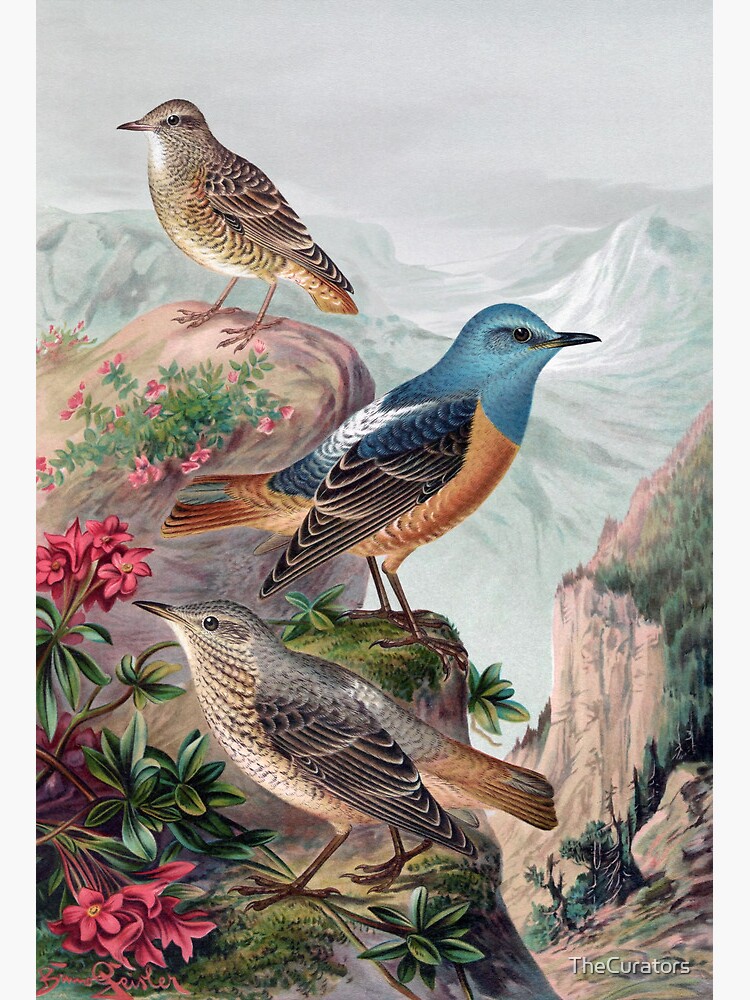This illustration, reminiscent of a John James Audubon piece, depicts three birds perched on a tan rock ledge adorned with pink tubular wildflowers and green leaves. The highest bird, perched on the topmost ledge, is a tan bird with a cream-colored neck and underbelly, looking majestically to the left. Below, on a lower ledge, is a blue bird with a blue head, face, and rump, brown underbelly, and tail feathers, facing to the right. Further down, another bird with grayish and brown feathers and a brown tail is also facing to the left. Adjacent to this scene is a sheer cliff with jagged pine trees growing in its crevices. In the background, faintly visible are snow-capped mountains that fade into a gray sky. The artwork is signed in red at the bottom left, with an indistinct name possibly reading “Chester” or “Lawler,” and a watermark on the bottom right states the curators' ownership rights.